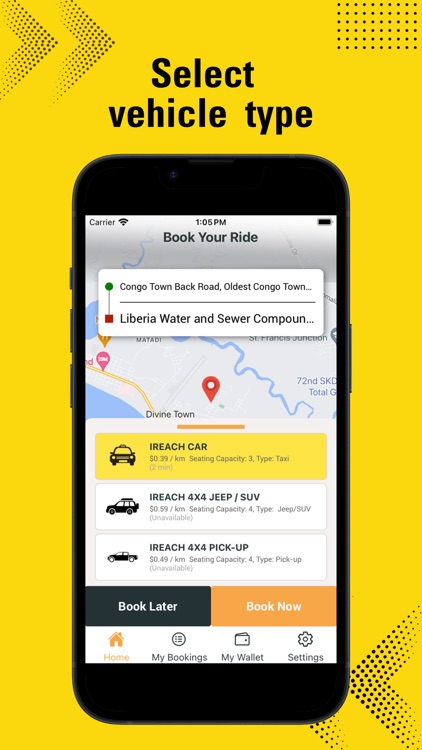This illustration depicts a smartphone showcasing a company's ride-booking app. The top section of the screen features a yellow background with the header text "Select Vehicle Type." Below this title, the smartphone display is prominently visible, with the app interface illustrating a route from Congotown Black Road to the Liberia Water and Sewer Compound. Users can choose their preferred vehicle type from options such as a car, truck, or SUV. Once the selection is made, the interface displays two orange buttons at the bottom, labeled "Book Later" or "Book Now," allowing users to schedule their rides conveniently. The detailed and vibrant design highlights the app's user-friendly functionality and essential features.